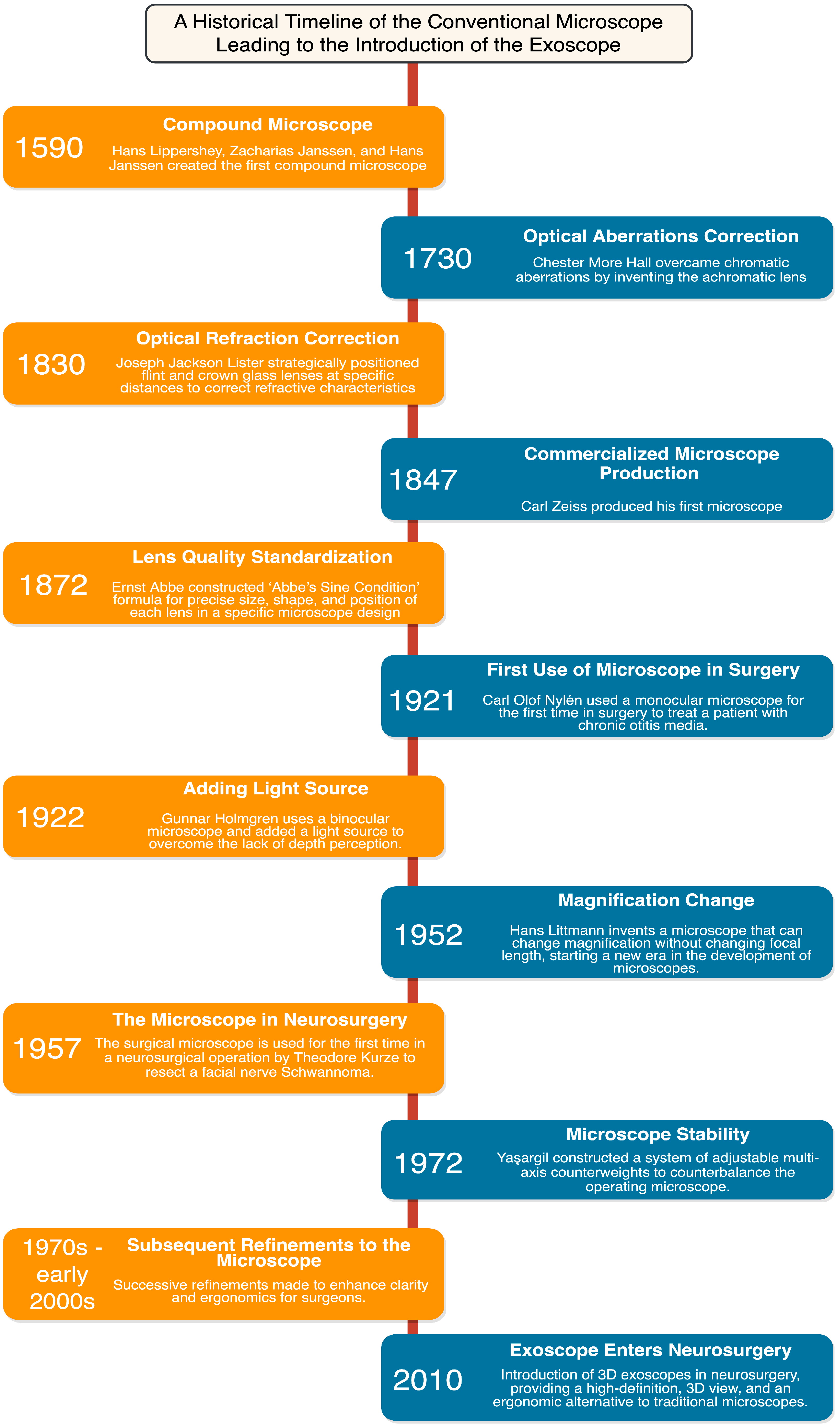The image displays a detailed vertical historical timeline chart titled "A Historical Timeline of the Conventional Microscope Leading to the Introduction of the Exoscope" against a tan background with black text. A red line runs down the center of the chart, with alternating orange tabs on the left and blue tabs on the right, each containing historical milestones and dates, accompanied by descriptive texts. Starting from the top, it highlights key developments: 1590 - Creation of the first compound microscope by Hans Lippershey, Zacharias Janssen, and Hans Janssen; 1730 - Correction of optical aberrations; 1830 - Correction of optical refraction; 1847 - Commercialized production of microscopes; 1872 - Standardization of lens quality; 1921 - First use of microscope in surgery; 1922 - Introduction of an integrated light source; 1952 - Advancements in magnification change mechanisms; 1957 - Microscope application in neurosurgery; 1972 - Improved stability of microscopes; 1970s to early 2000s - Subsequent refinements; and finally, 2010 - Introduction of the exoscope into neurosurgery, offering high-definition 3D views and ergonomic benefits. This academic infographic is suitable for educational purposes, such as a science class or a scholarly presentation.